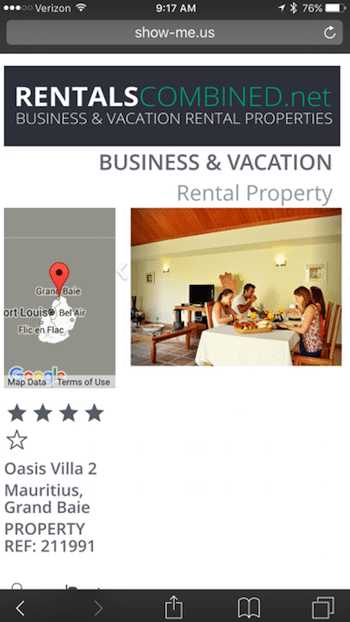The image showcases a mobile interface with various elements occupying different sections of the screen. At the top, there's a dark gray status bar displaying essential phone icons: three filled white circles on the left, two white-outlined circles, the Verizon logo, a Wi-Fi signal indicator, the time (9:17 AM), a paper airplane symbol, two right-pointing triangles with two horizontal lines underneath them, and finally a battery icon showing 76%.

Below the status bar, a lighter gray segment features the URL "show-me.us" and an icon of a partial circle with an arrow pointing to the right.

Further down, another gray bar includes the text "rentals," and underneath it, there is a vivid green label that reads "combine.net." The next segment has white text saying "business and vacation rentals and property." Directly below, the text repeats in a similar format: "business and vacation rental property."

The left side of the screen displays a Google Map with the Google logo occupying the bottom corner, indicating location details. On the right side, there is an image of a dining room where people are seated at a table, suggesting a social or meal setting.

Beneath the map, four gray stars are followed by a fifth star outlined in gray, and the label "Oasis Villa 2, Mauritius Grand Baie Property Ref 211991" identifies the property. 

At the very bottom, a dark gray navigation bar contains icons: an arrow pointing left, an arrow pointing right, a piece of paper icon with an arrow pointing upwards, an open book icon, and a stacked squares icon, likely representing various app functionalities or actions.